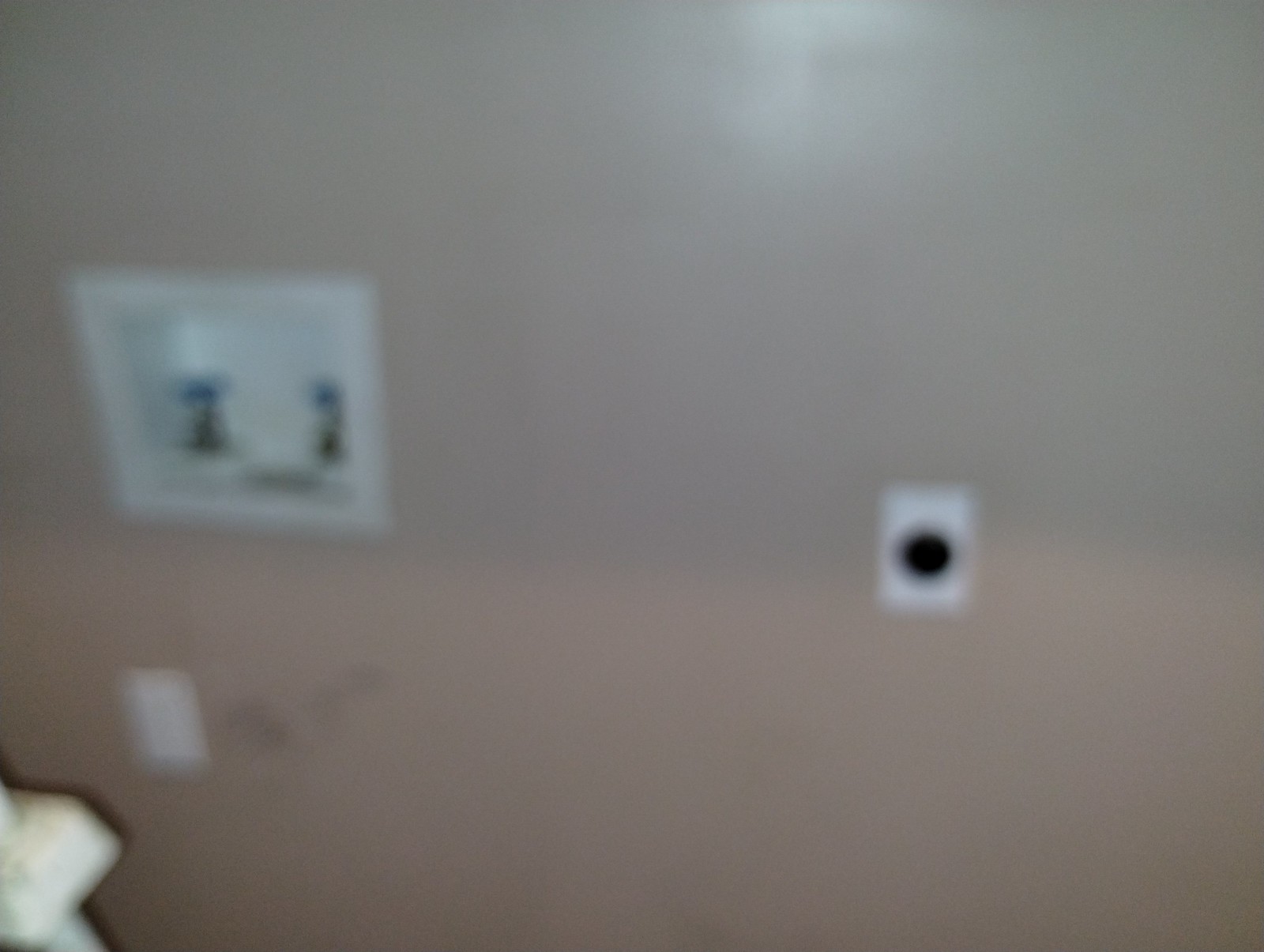The image appears blurry but provides an intriguing glimpse into a room, possibly a laundry area. The walls seem to be painted in two distinct shades or are subjected to varying shadows, with the bottom half displaying a peachy-brown hue and the top half resembling a grey-brown tone, possibly due to different paint colors or lighting effects. A light source positioned near the top center casts a soft white glow on the upper part of the wall, enhancing the greyish tint.

Towards the middle-right side, there is a white rectangle featuring a black circle at its center, potentially an electrical outlet or switch. To the left, a white square appears to frame a recess in the wall, housing two grey-silver valves with blue tops, possibly water hookups for a washer or dryer, indicating that this could be a laundry room. Below these valves sits another white rectangle, likely an additional outlet. The bottom left corner of the image shows a white, slightly dirty or dingy object, possibly fabric or trash. The overall blurriness of the image adds a layer of uncertainty to these observations.